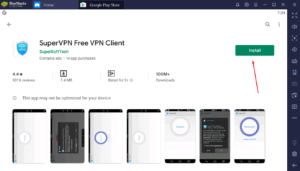The image depicts a webpage with a sleek, modern design featuring a black border at the top and along the right side. The main background of the page is white, providing a clean and contrasting backdrop. At the top of the page, a logo with yellowish and green hues is displayed, followed by a sequence of blue and white icon symbols, each accompanied by text.

In the top right corner, a cluster of icons and interactive buttons is visible, extending down the black border on the right side, offering additional functionality and navigation options.

The center section of the image is dominated by a prominent blue shield icon located on the left. To its right, bold text reads "Super VPN - Free VPN Client." Adjacent to this text is a noticeable green "Install" button, emphasized by a red arrow pointing directly beneath it for easy visibility.

Below the blue shield icon, there are star ratings and possibly user reviews, enhancing credibility. The bottom section of the page showcases various app screenshots, illustrating the app's interface and features in action. The overall layout is user-friendly, directing focus towards the essential elements of the webpage and the application it promotes.